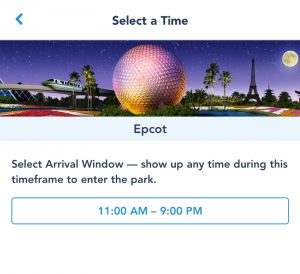This image depicts a selection screen for planning a visit to Epcot. The background is predominantly white, with the prominent text "Select a Time" in black at the top center. In the top left corner, there is a blue arrow icon.

The center of the image features a digitally rendered artistic representation of Epcot. Dominating the artwork is the iconic geodesic sphere, appearing in textured hues of gray, pink, gold, and orange, suggesting a scene set at sunset or nighttime. To the right of the sphere, a full moon is visible in the sky.

The artwork also includes the Eiffel Tower, surrounded by trees, and a sleek monorail traversing the scene, all set against a landscape that includes a serene pond and vibrant ground colors. Beneath this illustration, a light blue banner prominently displays the word "Epcot."

Below this banner, on a white background, black text instructs visitors to "Select arrival window – show up any time during this timeframe to enter the park." Further down, a thin blue rectangular border encloses a selection area with white inside. The available time slot, "11 a.m. to 9 p.m.," is displayed in blue characters.